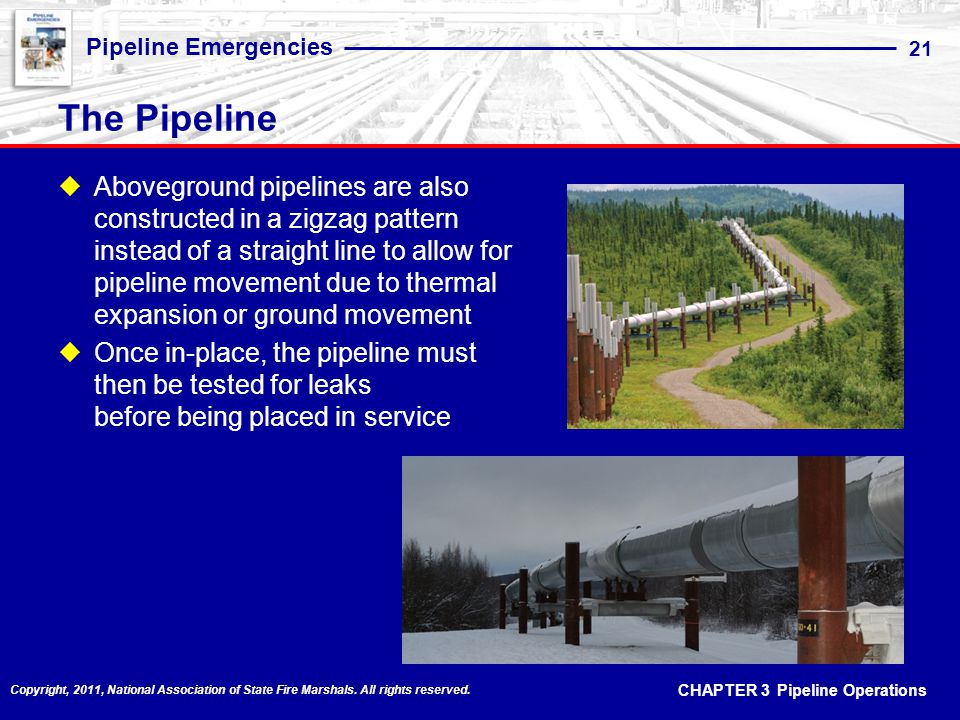This detailed image poster titled "Pipeline Emergencies" features a comprehensive overview of pipeline operations and safety measures. The title "Pipeline Emergencies" is prominently displayed in blue lettering at the top, accompanied by a number 21 at the far right end. Directly below, the subtitle "The Pipeline" is underscored by a red stripe.

The background of the poster is a deep blue, with important information highlighted in two yellow diamond-shaped bullet points positioned on the left side of the image. The first bullet point, written in white text, reads: "Above-ground pipelines are also constructed in a zigzag pattern instead of a straight line to allow for pipeline movement due to thermal expansion or ground movement." This is visually supported by an image to the right showing an above-ground pipeline arranged in a zigzag pattern amidst a lush, green landscape with a blue sky and mountainous backdrop.

The second yellow diamond bullet point states: "Once in place, the pipeline must then be tested for leaks before being placed in service." This point is complemented by a close-up image below, depicting a section of the pipeline supported by posts, set in a snowy environment with trees and a white sky in the background.

Additional details at the bottom of the poster include a copyright notice reading, "Copyright 2011, National Association of State Fire Marshals, All Rights Reserved," located at the bottom left corner in white text. On the bottom right, in similar white text, it says, "Chapter 3, Pipeline Operations."

The overall design juxtaposes the instructional yellow bullet points on the left with corresponding pipeline images on the right, creating an informative and visually engaging layout that details the construction and testing protocols of above-ground pipelines.